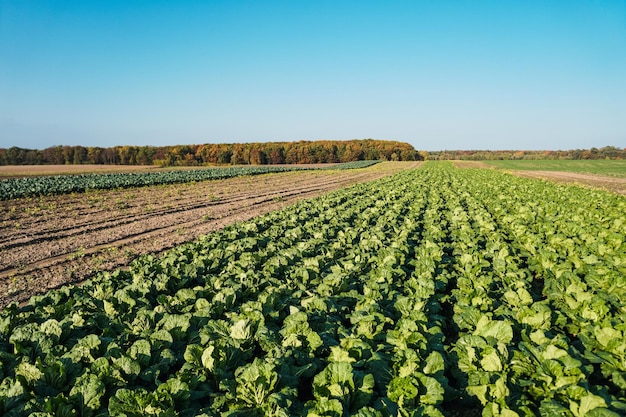Beneath a vast, radiant blue sky dotted with a few wisps of white clouds, stretches an expansive agricultural landscape. The foreground is dominated by a meticulously plowed field, neatly segmented into perfect rows of vibrant green leafy plants that are thriving. To the left, adjacent fields reveal various stages of growth: some with young sprouts bravely emerging through the soil, while others showcase more mature plants flourishing under the sun. In the distant background, a grand row of towering, lush green trees stands as a natural boundary, enhancing the bucolic beauty of the scene. The entire vista encapsulates the essence of a bountiful and well-tended farmland.